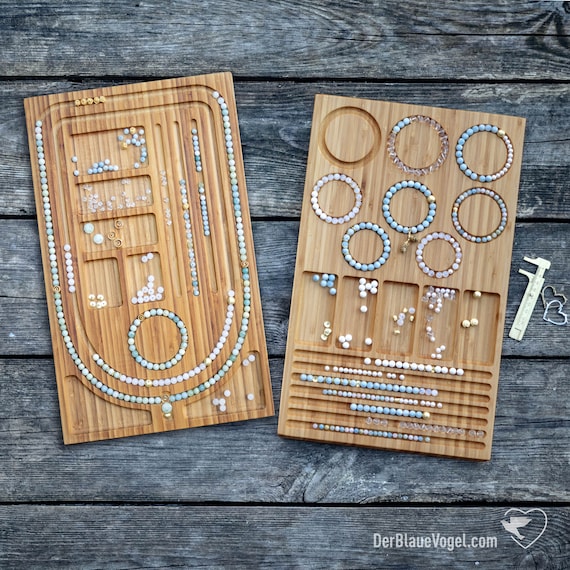This top-down photograph captures a detailed beading kit set against a light gray wooden plank background, with the planks running horizontally. The kit, designed for creating bead jewelry, consists of two vertical rectangular wooden boards. Each board features meticulously carved grooves and indentations filled with an assortment of beads.

On the left board, there are long, thin grooves around the perimeter, numerous smaller indentations, circles, and rectangles, all populated with beads. The patterns suggest spaces for threading necklaces and bracelets. The beads vary in color, including white, light blue, yellow, pink, and pearl-like shades.

The right board contains circle patterns and a mix of rectangular and narrow indentations, similarly filled with colorful beads. Additionally, it houses a white measuring caliper on the far right side, and two heart-shaped charms. Notable is a logo on the bottom that features a heart with a dove inside and the inscription "Der Blau Vogel" or "derblauvogel.com." This kit appears to be highly organized and designed to assist in the creation and precise measurement of beaded jewelry.